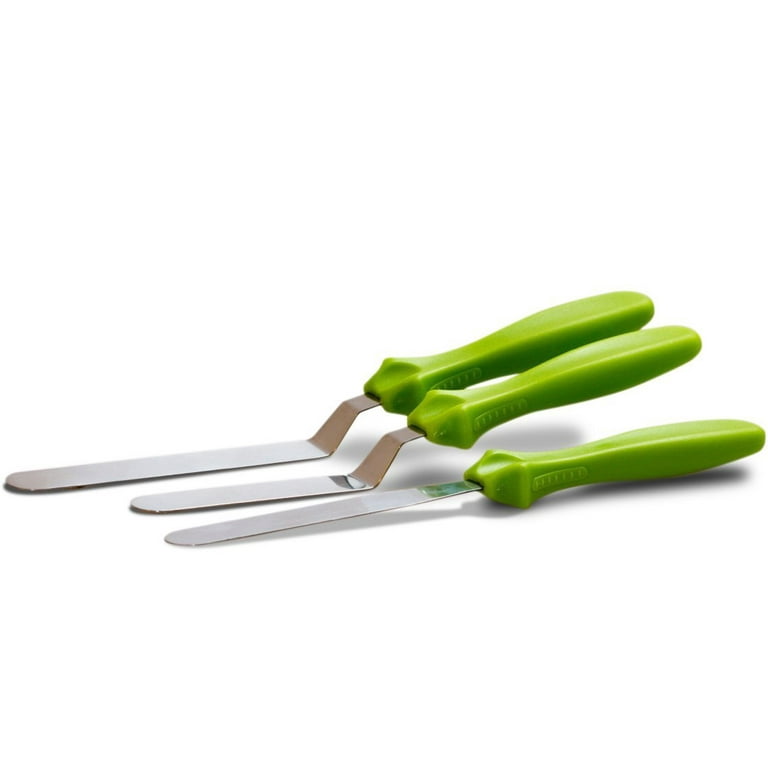The image is a product or catalog photo of three culinary utensils, captured against a clean white background, likely with overhead lighting that casts subtle shadows underneath each tool. All three utensils feature lime green handles designed with ridges for ergonomic thumb placement, enhancing grip for ease of use. The functional parts of the tools are made of shiny silvery metal, most probably stainless steel. 

The first utensil, positioned closest to the camera, resembles a knife with an oblong, rounded metal blade that remains straight and unserrated. The second utensil, lying in the middle, is a shorter spatula, characterized by its flat metal surface that bends slightly downward into a flatted end, ideal for scooping. The final tool in the background is a longer spatula, designed similarly to the second one but larger in size, possibly intended for tasks requiring greater reach or leverage. Despite slight variations in lengths and forms, the metal parts of all three utensils are thin and flat, optimized for their respective cooking or baking purposes.